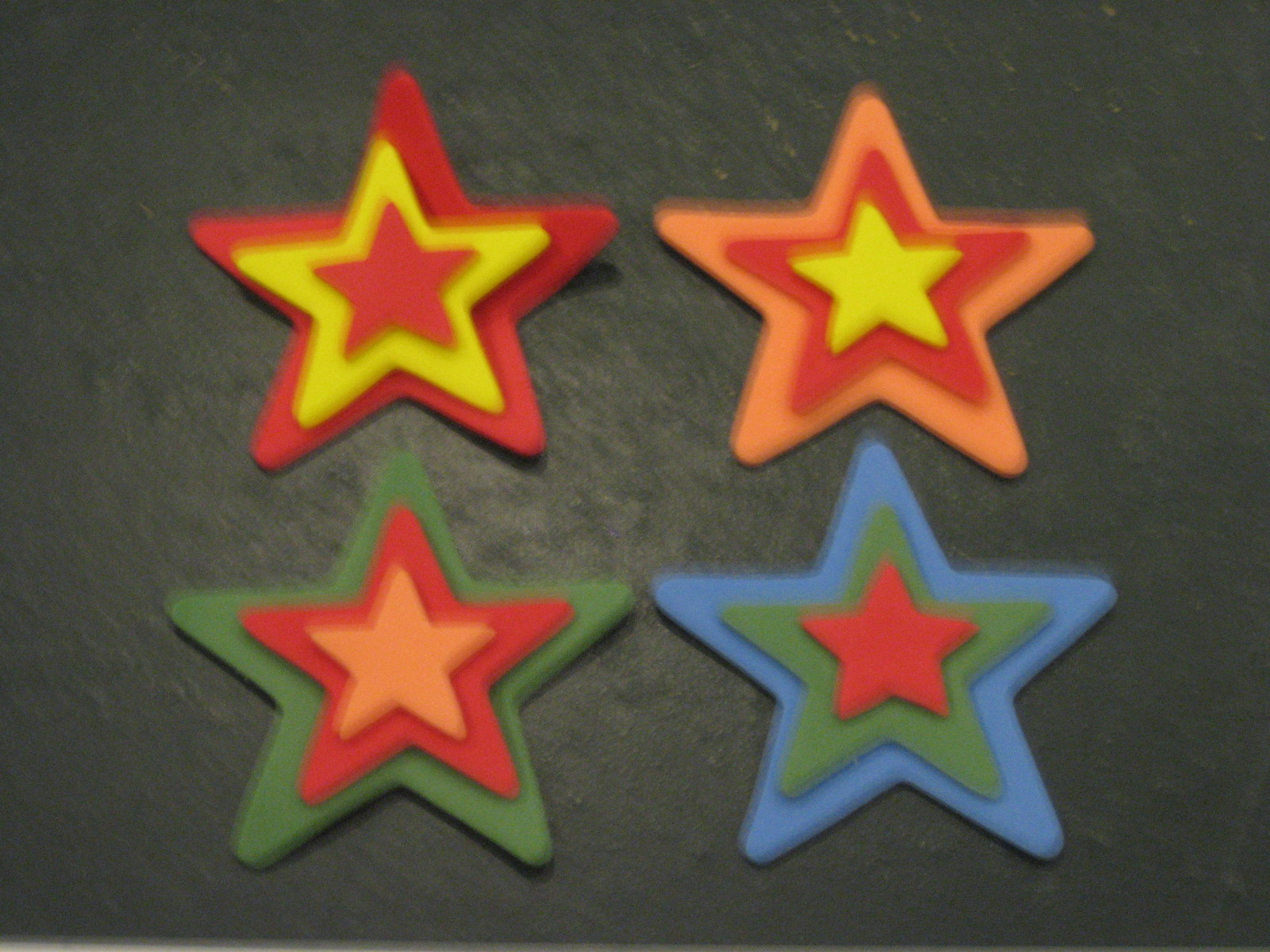The image is a slightly blurry photograph depicting four colorful, multi-layered stars arranged against a black backdrop. The stars are stacked in a 2x2 grid, with two on the top row and two on the bottom row. Each star comprises three nested layers, each smaller than the one beneath it, in varying color combinations:

1. The top-left star has an outer border of red, a middle layer of yellow, and an innermost layer of red.
2. The top-right star features an orange outer border, with a central red layer and an innermost yellow star.
3. The bottom-left star's outer layer is green, the central layer is red, and the smallest inside layer is orange.
4. The bottom-right star has a blue outer border, a central green layer, and a red innermost star.

The stars appear to be crafted from a material such as Play-Doh, paper, or similar and are positioned symmetrically two on the top and two on the bottom. Each layer within the stars is meticulously detailed and colorful, adding a vibrant contrast against the mottled black background.